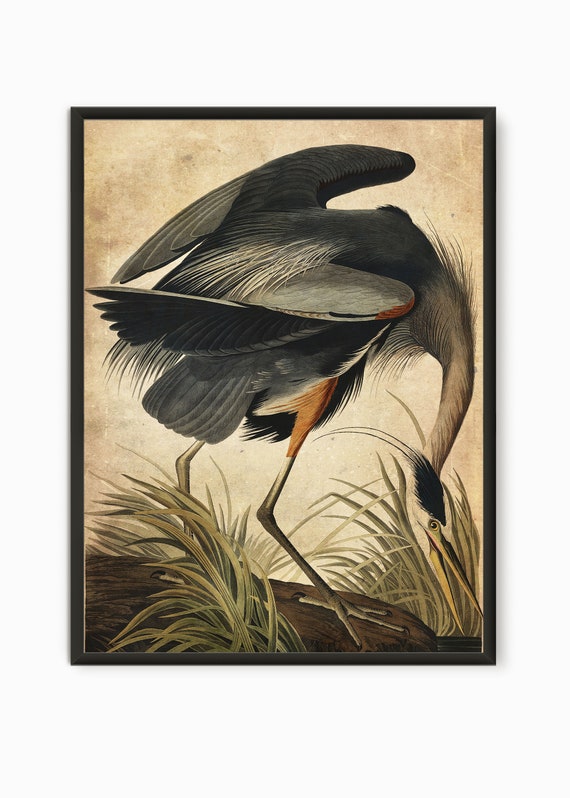This is a colorful framed painting of an impressive aquatic bird, possibly a stork or a crane, presented in portrait style against a light brown, almost dirty beige background. The bird, which is mostly gray and black with accents of white feathers, has especially long and slender legs with a hint of orange near the top. Its extended leg appears to be embedded in dirt, surrounded by green grass and plant stalks.

The bird boasts a striking long neck that curves downward, leading to a long, sharp beak with yellow highlights. The neck itself is white, adding a contrast to the predominantly gray and black body. Its head features large eyes and distinctive black feathers, with a quill-like crest. The wings, primarily black with gray and white, have subtle orange touches at the tips, adding a pop of color.

Set against a backdrop evoking a near-aquatic environment, though water isn't visible, the scene suggests the bird is poised on a bank, ready to skewer fish with its pronounced beak. The overall composition, framed in black, hangs on a white wall, capturing the essence of this majestic bird in its natural habitat.